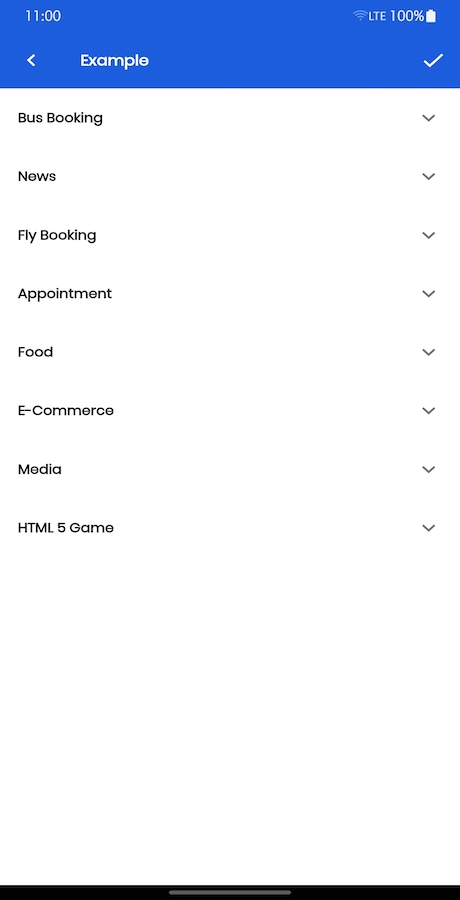The image features a white background. At the top, there is a prominent blue rectangle displaying an example interface. On the left side of this blue box, there is a left-pointing arrow and the text "11:00 AM." On the right side, various status indicators are shown, including LTE signal strength and a battery icon indicating 100% charge, along with a white checkmark.

Below this blue section, the white background continues with a list of categories, each accompanied by a down arrow on the right side. The categories are sequentially listed as:
- Bus booking
- News
- Fly booking
- Appointment
- Food
- E-commerce
- Media
- HTML5 game

Each category title is followed by its respective down arrow, indicating that they are likely dropdown menus or expandable sections.

At the bottom of the image, there is a small black rectangle with a thin gray line running through it, situated on the white background. This appears to be a navigation or menu element.

Overall, the layout is clean and minimalistic with a clear distinction between the blue header section and the white content area below, organized with a series of categorized titles and navigation prompts.